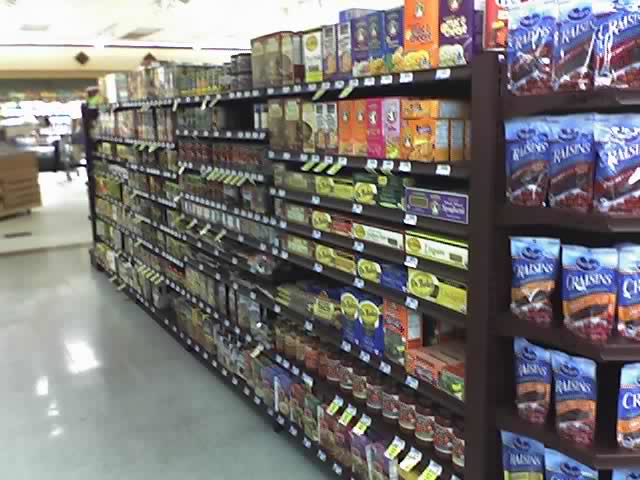This photograph captures an aisle inside a supermarket, viewed from a slightly angled perspective with the display racks prominently displayed on the right side. The aisle floor is shiny, displaying a greenish hue, and you can see the reflection of an overhead light source. The shelves are black and stocked with various items, with a notable section dedicated to craisins which are stored in bluish bags featuring a clear center to showcase the contents. These craisins bags have a blue banner with red and orange accents toward the bottom.

The top shelves appear to house cereals, while the second shelf from the bottom contains jars of pasta sauce. To the left of the craisins, there is a mix of products that could include cereals, pasta, boxed potatoes, or macaroni and cheese. Owing to the image’s blurry quality, finer details of these items are hard to discern. In the background, more shelves are visible but also blurred, reducing the clarity of the products displayed further down the aisle. The roof above is white, and to the left-hand side in the background, there is a suggestion of another store section, possibly a deli department.